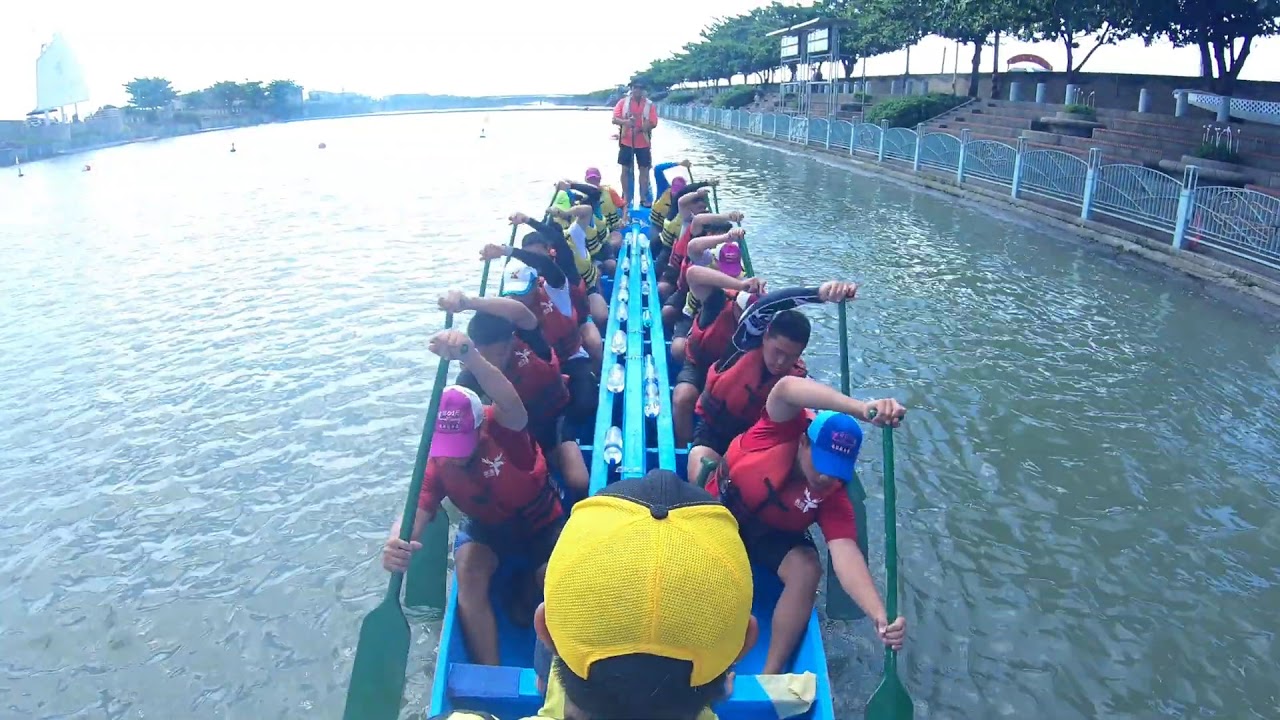The photograph captures a vibrant scene of a rowing team in action on a clear, sunny day. The team is navigating a large blue rowing boat, with fourteen rowers (seven on each side) synchronized in their strokes, lifting their green oars high above the water. Each rower is dressed in a red shirt with a logo, possibly featuring a deer, and they are all equipped with orange life jackets and various colored hats, including pink, blue, and white. At the back of the boat stands an instructor in a neon vest, possibly holding a stopwatch, while at the front, another leader with a yellow cap commands the team. They are rowing on a wide river, bordered on the right by a fence, steps, and a line of trees. The water has a glare, suggesting it is a clear, bright day, with the surrounding cityscape enveloping the tranquil river setting.